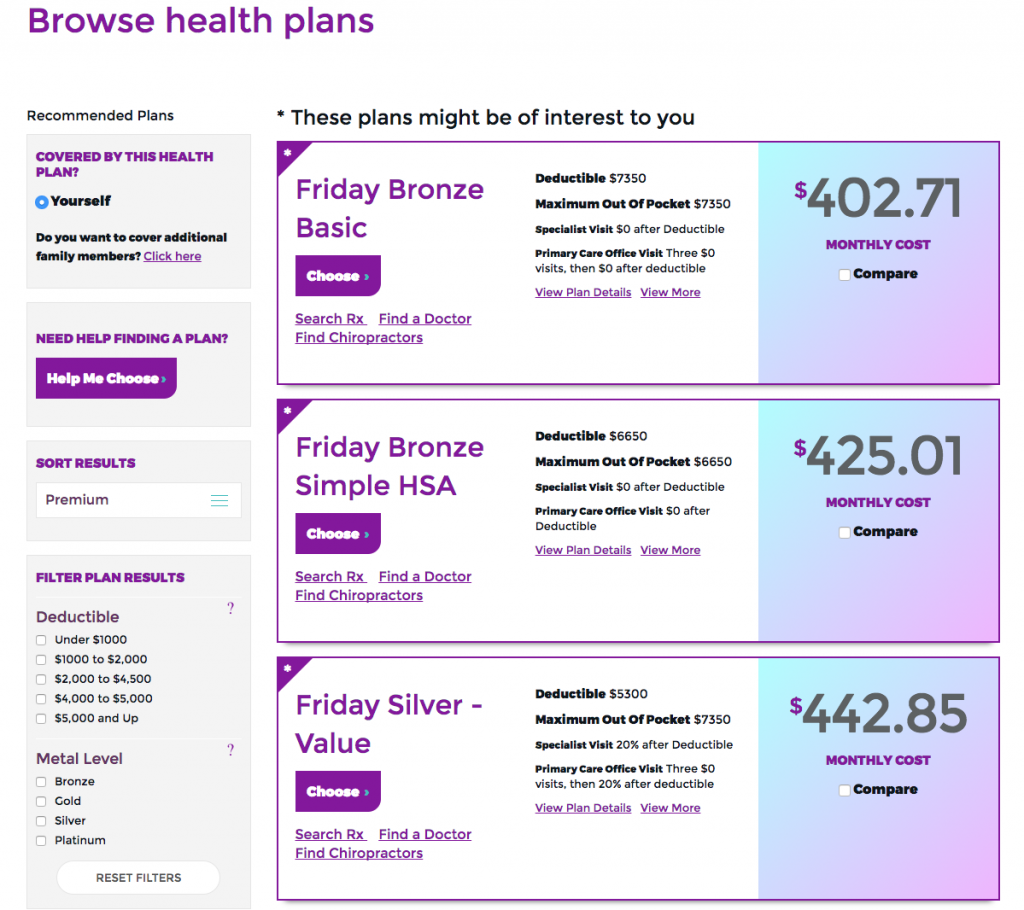This image is a screenshot from a website designed to compare and contrast various health plans. At the top of the page, a violet-colored header reads "Browse Health Plans," indicating the main function of the site. The layout is divided into two distinct sections.

On the left quarter of the page is the "Recommended Plans" section. Here, the first item mentions "Covered by this health plan," with the option "Yourself" pre-selected using a blue radio button. Below this, there is a prompt asking, "Do you want to cover additional family members?" with a clickable link in purple text that says "Click here." Additionally, users seeking further assistance are invited to click a rounded rectangle button labeled "Help me choose." This section also provides options to sort results by premium and filter plans based on deductibles ranging from under $1,000 to above $5,000. Furthermore, users can filter by metal level—Bronze, Silver, Gold, and Platinum—and have the ability to reset these filters.

The remaining three-quarters of the page is devoted to the "These Plans Might Be of Interest to You" section. Highlighted here are three plans from "Friday Health Plans": 

1. **Friday Bronze Classic** - Monthly cost of $402.71
2. **Friday Bronze Simple HSA** - Monthly cost of $425.01
3. **Friday Silver Value** - Monthly cost of $442.85

Each plan's details, such as its name and monthly cost, are prominently displayed, aiding users in making informed decisions.